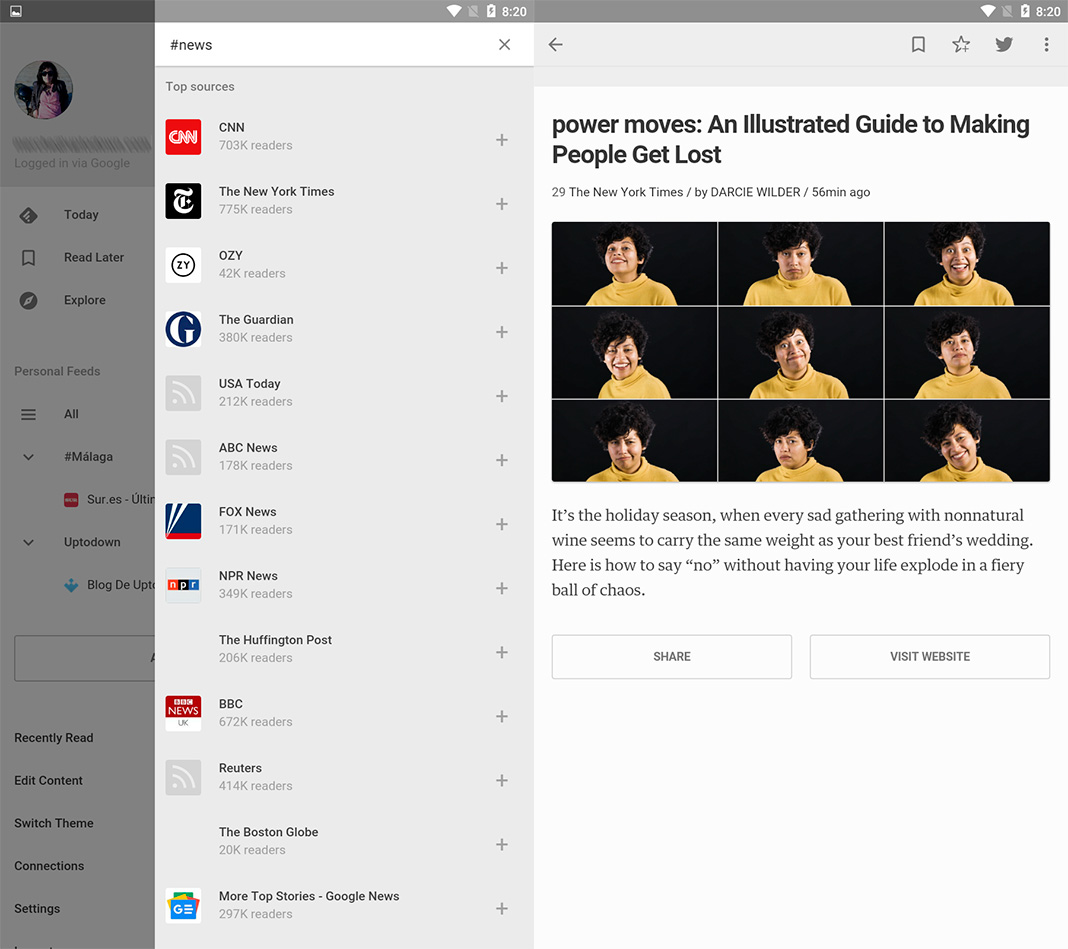The image appears to be a screenshot of a news website displayed on a laptop. At the top right of the screen, the laptop's status bar shows it is 8:20 AM, with full Wi-Fi bars, a shaded-out bell icon, and a battery icon. 

In the middle right section of the screen, a prominent article is featured. The article title reads, "Power Moves in Illustrated Guide to Making People Get Lost," displayed in bold black text. The byline below the title states "29, The New York Times / by Darcy Wilder, 56 minutes ago."

The article is accompanied by a square collage comprising nine boxes, each showing different facial expressions of the same individual. The expressions are arranged as follows:
- **Top Row**: Happy, Sad, Very Happy
- **Middle Row**: All Happy
- **Bottom Row**: Sad, Sad, and Happy

Beneath this collage, there are two rectangular buttons labeled "Share" and "Visit Website."

On the left side of the screen, a vertical list of popular news outlets can be seen. The listed news sites are: CNN, New York Times, OZ, The Guardian, USA Today, ABC News, and Fox News.